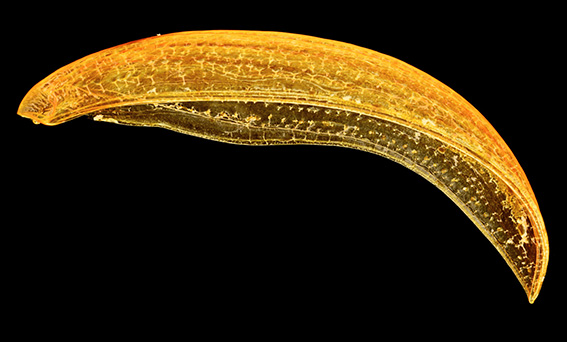The image features a bright, golden-orange crescent-shaped object set against a black background. The object resembles an arc, similar to an orange slice or an inverted canoe with both ends pointed downward. The exterior of the object is vividly orange, transitioning into yellow, while the interior contains intricate specks or dots, resembling the pulp of a fruit. The details inside appear almost microscopic, with the tiny specks standing out in bright yellow. The transparent-like quality and elongated shape of the object suggest it could be a magnified view of a microorganism, showcasing fine vessel-like structures within its body. The overall appearance is decorative and intricate, with carvings or patterns that enhance its visual complexity.